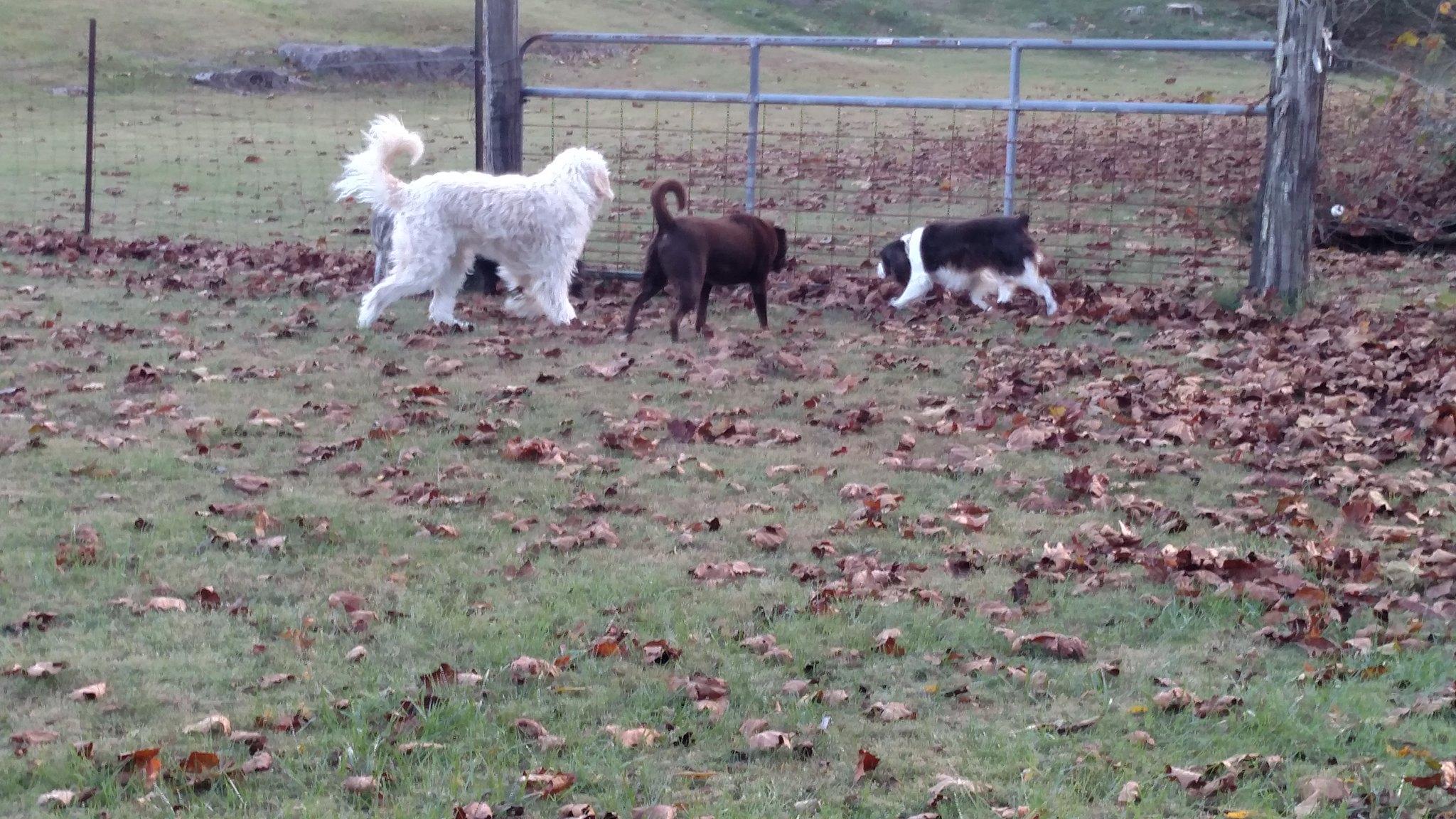The image depicts a farmyard in autumn, characterized by a metal gate similar to one used for a pen. The gate, designed with vertical rods and cross-wires, stretches across the back of the yard and includes a sliding mechanism to access another field. The ground is a dull green, overlaid with numerous fallen brown leaves, suggestive of the fall season. Three dogs are in the yard, near the gate. The first, a large white dog with long fur, resembles a St. Bernard. The second, a brown, stocky dog with its tail curved upwards, has its face turned away. The third dog, smaller and likely a mixed breed with hound characteristics, has a black back, white legs, and black ears. All three dogs are positioned as if interested in the gate, possibly awaiting access to another area.